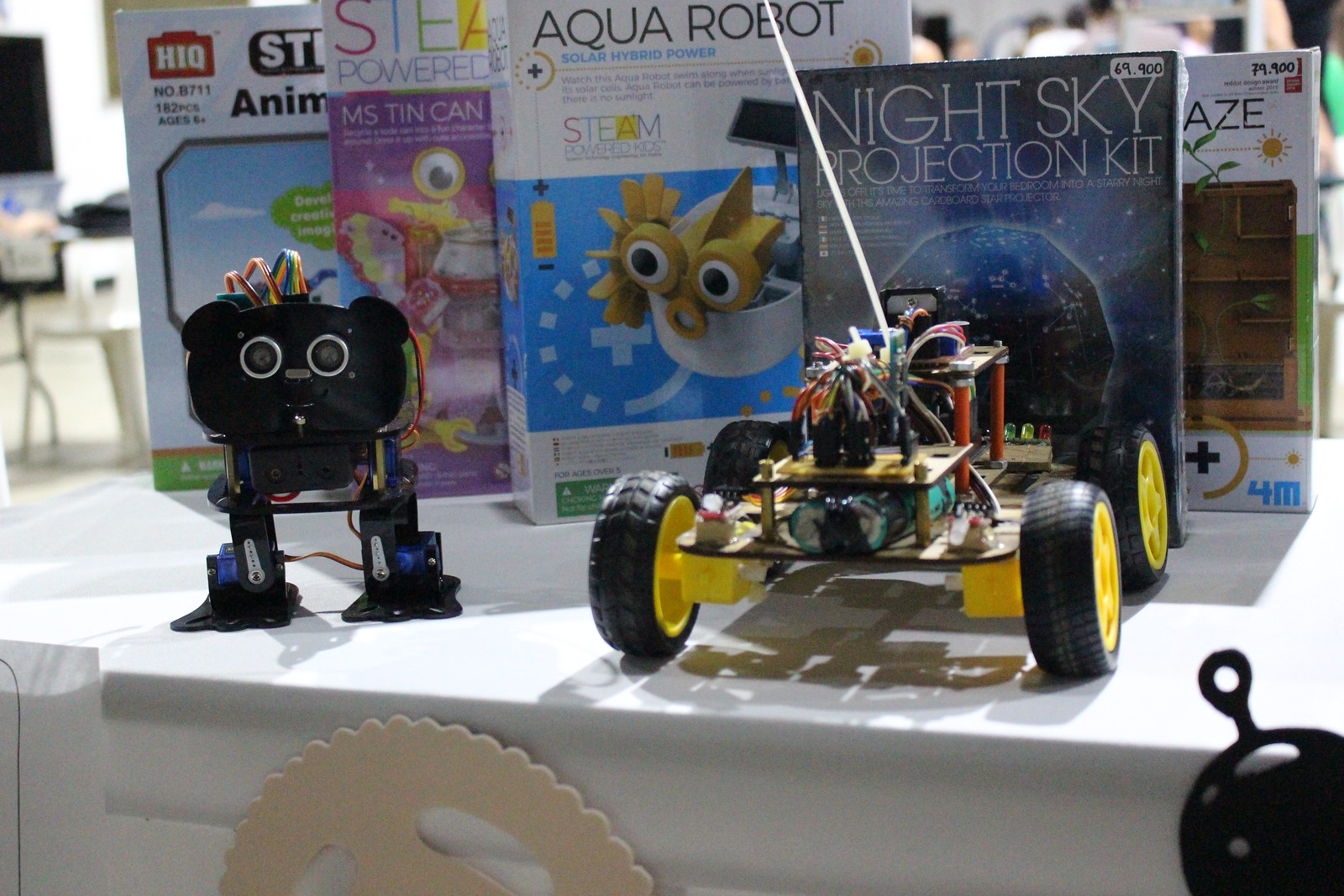On a white tablecloth-covered table, this indoor photograph features two handmade robotic toys prominently displayed in front of a series of gadget kits. To the left, there's a black bear-shaped robot made from a combination of electronic components, including wires protruding from its head and sides, and small robot legs with interconnecting wires. It has lens-like eyes and a handcrafted feel. To the right is a remote-controlled car without a traditional body, instead featuring exposed circuit boards, LED lights, batteries, and a tangle of wires, giving it an unfinished, DIY appearance. Behind these robotic toys are various boxed kits, including a "Night Sky Projection Kit" with an image of a globe, an "Aqua Robot Solar Hybrid Power" kit displaying a fish-shaped robot with a solar panel, and a "Growing Plant Maze Kit" for growing plants through a maze. Additionally, there are boxes labeled "Mistin Can" and an unreadable one, adding to the impression of a scientific or educational store display.